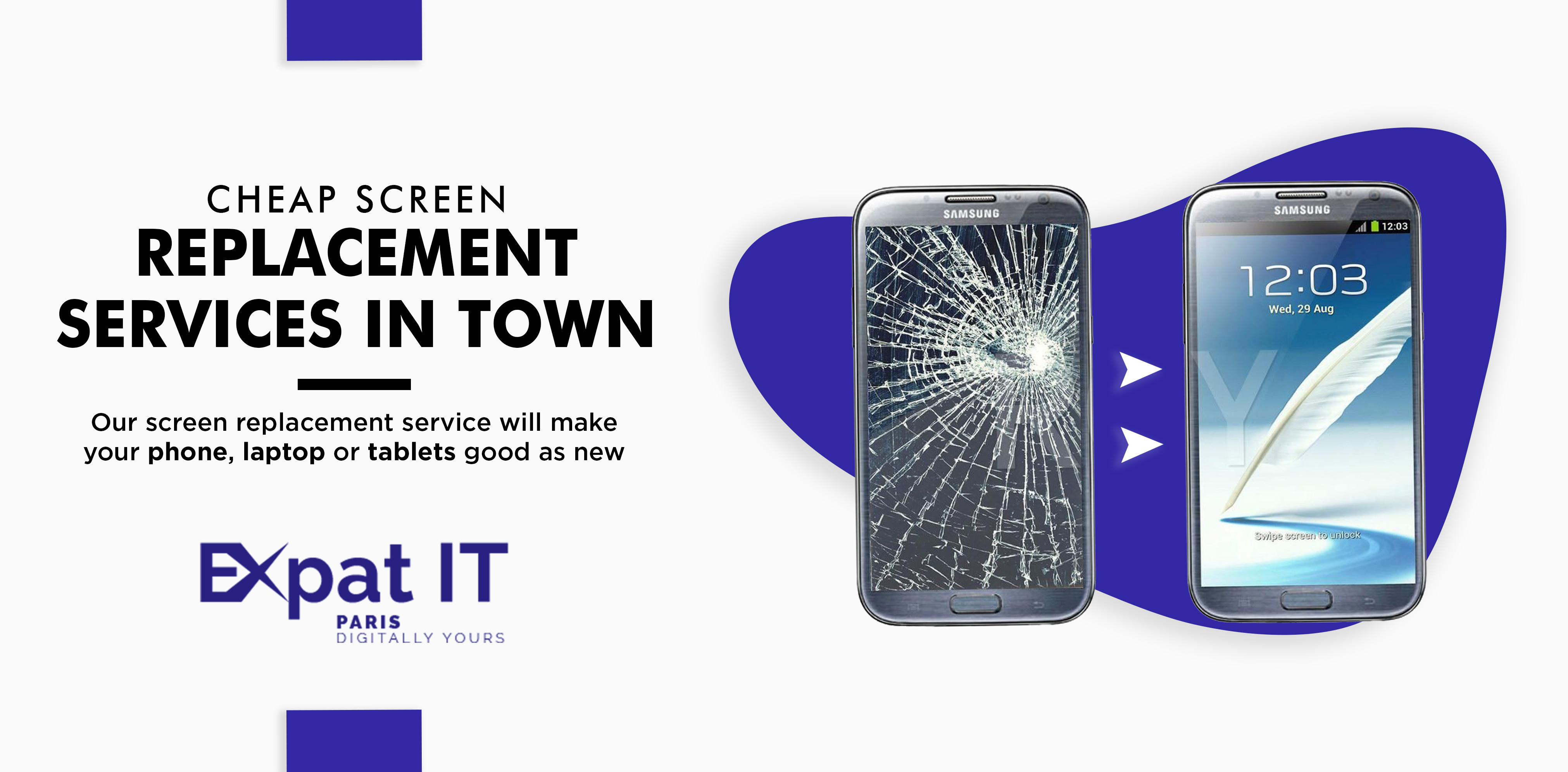The advertisement features a clean, mostly white background that puts the primary focus on the elements presented. On the right side, there are two Samsung phones – one with a completely shattered screen, and the other restored to perfect condition. The restored phone displays the time and date, "12:03 Wednesday, 29th August." Positioned behind the phones is a liver-shaped purple logo, adding a geometric, ovular backdrop to the image.

On the left side of the advertisement, a block of blue color highlights the text: "Cheap screen replacement services in town." Below this, in black text, it states, "Our screen replacement service will make your phone, laptop, or tablet as good as new." Further down, the company logo, "Expat IT Paris," and the tagline, "Digitally Yours," are displayed, followed by another blue block.

Additionally, purple rectangles adorn both the top and bottom of the advertisement, adding to the cohesive color scheme which includes shades of blue, purple, black, white, gray, and tan. The overall design indicates a professional screen replacement service, ensuring that devices like phones, laptops, and tablets will be restored to their original condition.